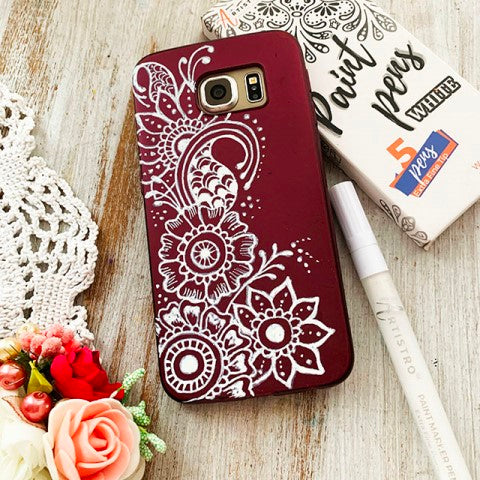In this indoor photograph, several items are arranged on a roughly finished wooden table. Centrally, there is a cell phone encased in a maroon cover adorned with intricate white floral designs, likely crafted using the white paint marker seen beside it. The phone case features two camera lenses on its back. Diagonally next to the phone is a white paint marker labeled "Artistro" and "paint marker." Nearby, a white box marked "paint pens white, 5 pens extra fine tip" suggests that this is part of a craft project. To the left of the phone, there is a white crocheted lace doily accented with a peach-colored rose, another red rose, pink beads, and some artificial berries. This arrangement provides a decorative and artistic setting on a wooden surface.